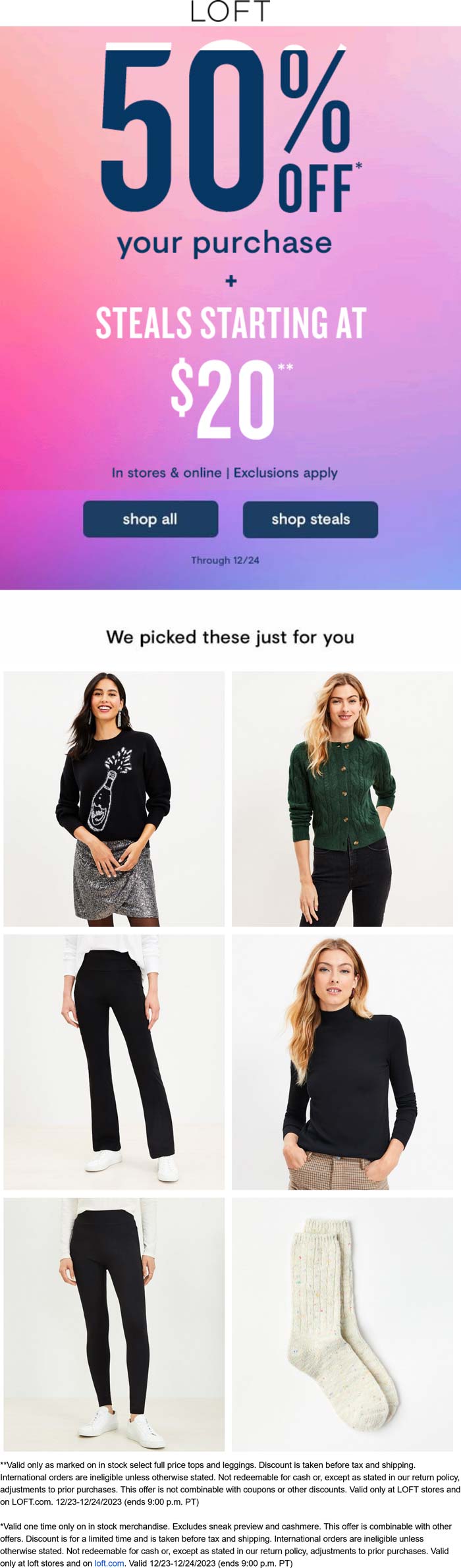This visually engaging advertisement features a white background with prominent branding at the top, denoted by the text "L-O-F-T" in a sleek gray font. Below the brand name is a large square with an eye-catching gradient that transitions from a soft pink at the top to dark pink in the middle, and culminates in a rich purple at the bottom. 

Dominating this gradient background, "50% off your purchase" is boldly stated in large purple font. Accompanying this, a white plus sign introduces additional offers, "steals starting at $20," providing an enticing call to action. 

Further details follow in black font beneath these promotional highlights: "in stores and online" with a small vertical line separating "exclusions apply." Two purple buttons with white font offer interactive options— "shop all" on the left and "shop steals" on the right, complemented by a note, "through 12/24," reminding customers of the sale's end date.

Below the promotional square, the advertisement transitions back to a white background with the tagline, "we pick these just for you," in black font. This section showcases two vertical rows of three curated product images. 

In the top left image, a Latina woman showcases her style in a black t-shirt paired with a silver skirt. Next to her, a blonde woman is seen wearing a button-up gray shirt and black pants. The middle left image features a pair of tightly fitted black pants, ideal for modern, sleek looks. On the middle right, the blonde woman reappears, this time styled in a sophisticated black turtleneck.

This detailed layout not only captures the viewer's attention but also seamlessly provides all necessary details to encourage immediate shopping action.